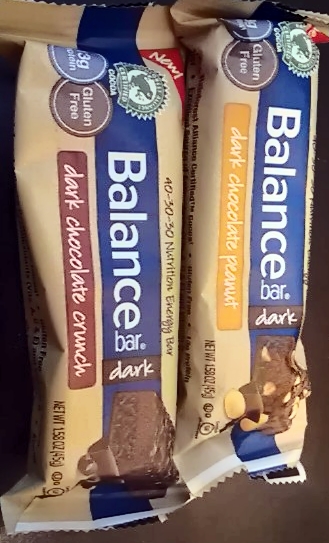This photograph features two packaged snack bars positioned vertically side-by-side, revealing their sides rather than their fronts or backs. Each bar follows a consistent design scheme with a tan background and a prominent blue stripe running vertically through the center.

The left snack bar displays a maroon rectangle near the bottom left corner. Inside the rectangle is the label "Dark Chocolate Crunch" written in white. Positioned centrally within the blue stripe is the brand name "Balance Bar" depicted in white letters. Further up the blue stripe is a black strip with the word "Dark" in white and an image of a piece of chocolate bar beneath it. Toward the top of the package, a green-outlined circle containing a green frog against a white background is present. Adjacent to this circle, a blue circle with white text and a brown circle with light brown text that reads "Gluten Free" are positioned on the left and right, respectively.

The right snack bar is identical in design, with the key difference being the maroon rectangle is replaced by a yellow rectangle. The yellow rectangle contains the label "Dark Chocolate Peanut" in white text.